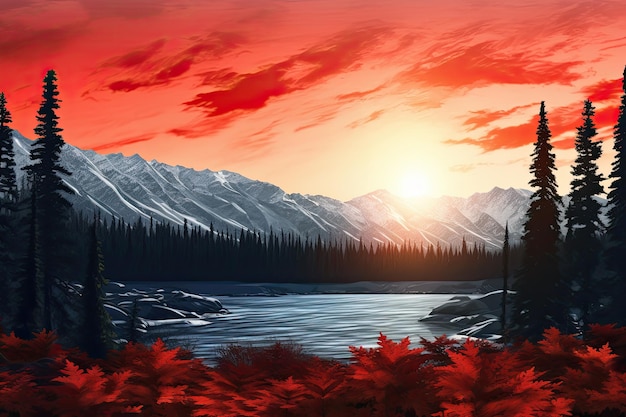This digitally-created anime-style painting depicts a serene mountain scene at sunset. The sky is awash with shades of red, blending into yellow where the sun sits just above the mountain ridge, casting a brilliant glow. Dark red clouds streak across the sky, adding depth to the twilight ambiance. The mountains are characterized by their plain gray rocky surfaces, with a light dusting of snow atop them. In the middle ground, a calm, gray-blue lake or river is flanked by a dense forest. Tall pine trees, both in the distance and closer to the viewer, frame the landscape. In the immediate foreground, vibrant red leaves are scattered, mirroring the deep hues of the sky and suggesting a setting in the fall. Rocks punctuate the shoreline, completing this tranquil autumnal scene.